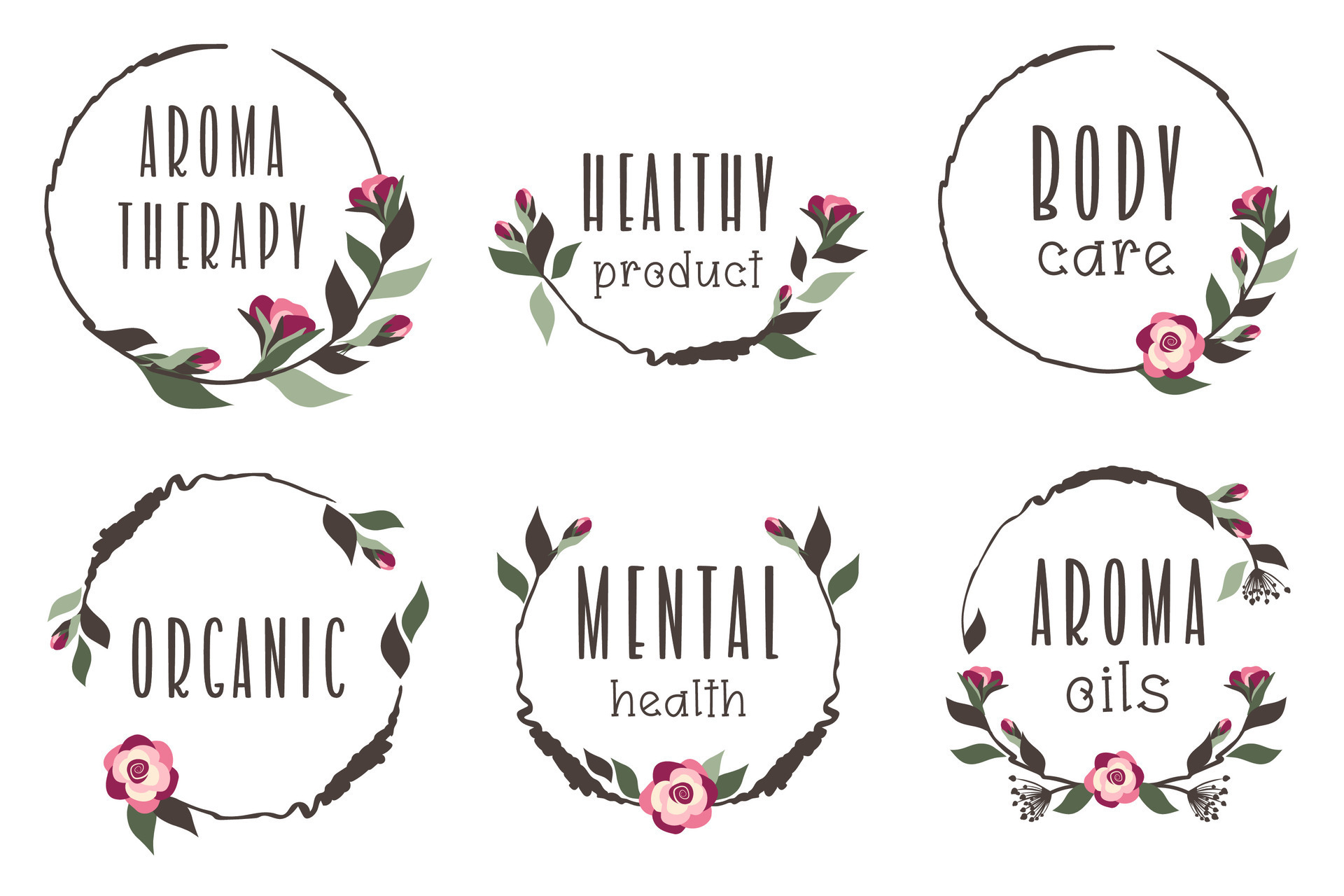The image is a digital poster featuring six distinct labels, each bordered by decorative floral designs. In the top left corner, the label reads "Aromatherapy" in dark brown capital letters, encircled by a ring of pink flowers, green leaves, and brown stems. Directly to the right, the words "Healthy Product" are displayed, also embellished with flowers and leaves forming an incomplete circle around the text. Continuing to the right, the label "Body Care" appears with a similar floral design.

On the bottom row, starting from the left, the label "Organic" is shown with a decorative circle of flowers and leaves. Next to it, the words "Mental Health" are encircled by the same type of floral arrangement. Finally, in the bottom right corner, the label reads "Aroma Oils," adorned with another intricate design of flowers and leaves. The background of the poster is white, and all texts are in a cute, comic-style font, giving a cohesive and aesthetically pleasing look. The overall structure suggests an advertisement for products related to aromatherapy, mental health, and body care, each label artistically highlighted by botanical elements.